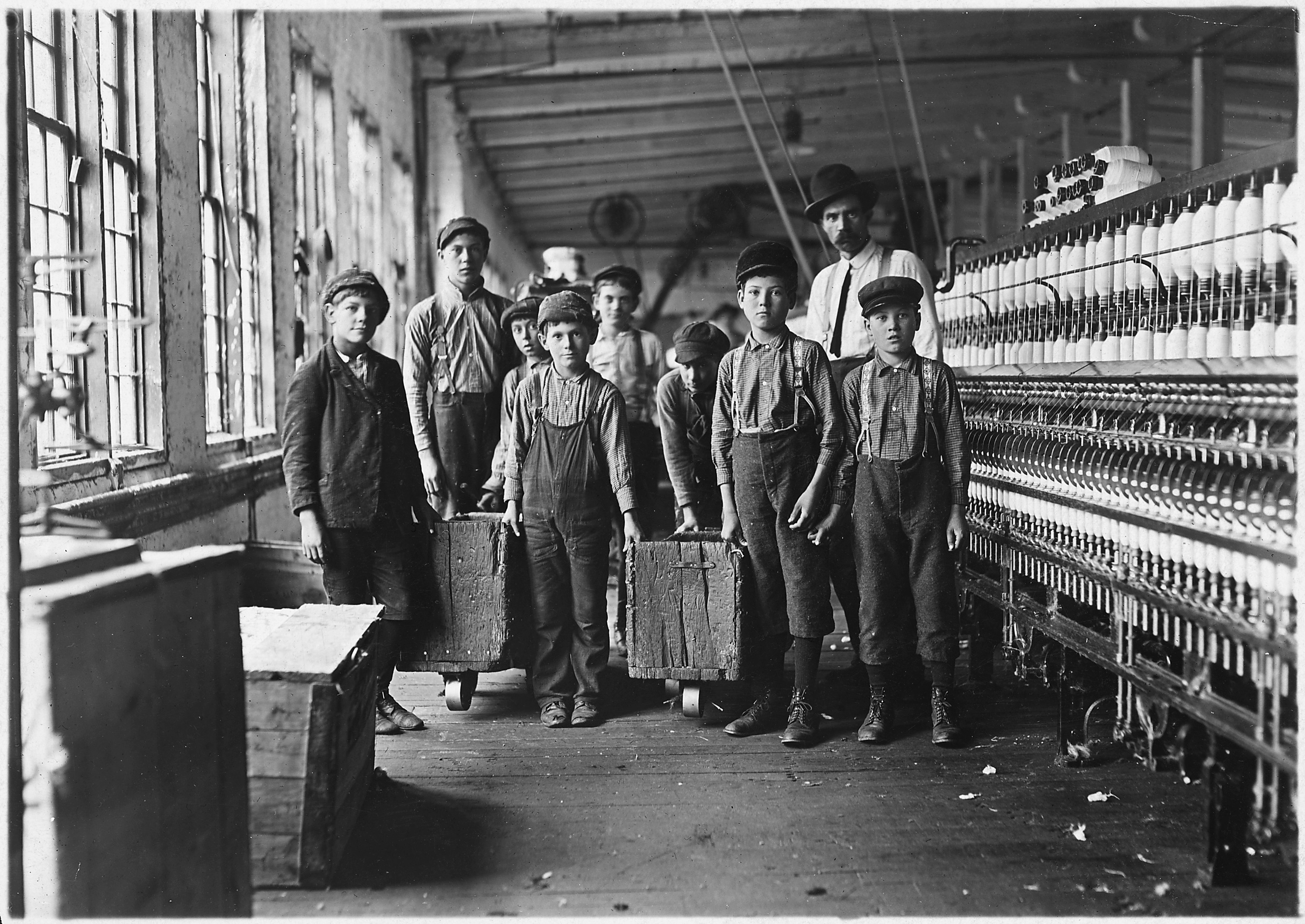This highly detailed black-and-white photograph appears to date back to the early 20th century and showcases a group of young boys in an industrial factory setting. The boys, who are the focal point of the image, are dressed in overalls, caps, and old leather shoes, suggesting a sense of poverty. They are holding large wooden trunks. In the background, a man with a mustache, wearing a white shirt, tie, suspenders, and a hat, stands observing the scene. The left side of the photograph reveals an industrial machine laden with yarn as well as wooden crates, with fabric pieces scattered across the floor. The left wall is lined with windows, allowing light to stream in and illuminate the room. To the right, an assembly line or some form of machinery is visible, loaded with various parts. The group seems to be posing intentionally for the photograph, encapsulating a moment in time that likely reflects the era when child labor in factories was commonplace.